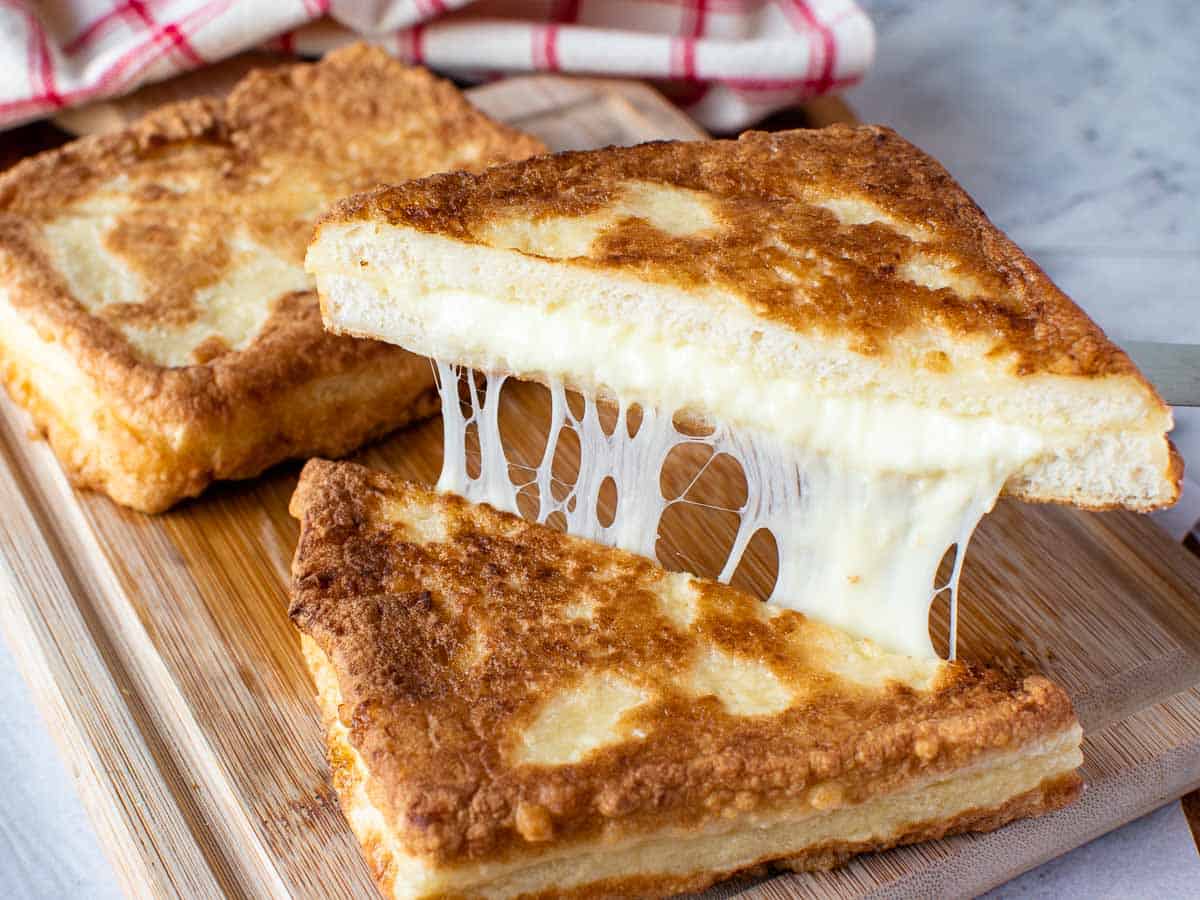In this detailed, close-up image, we see a vibrant and appetizing scene featuring two grilled cheese sandwiches displayed on a wooden cutting board with a shallow groove around its edge. The image is almost a perfect square in shape, and the composition conveys a homely, rustic kitchen vibe with a red and white checkered towel in the background.

One sandwich appears whole, showcasing its beautifully toasted, golden-brown crust with bubbly, crispy nooks and crannies, suggesting a generous amount of butter was used in the cooking process. The second sandwich, positioned closer to the viewer, is cut diagonally into two triangular halves. One of these halves is being lifted to reveal a mouthwatering cheese pull, with the creamy, white, and slightly melted cheese stretching tantalizingly between the bread slices. The cheese appears to be akin to Swiss, with visible holes and a smooth, luscious texture.

The bread crust is visibly crisp and perfectly browned, with some clear areas showing a less cooked surface, adding to the overall visual appeal. This setup on a marble countertop provides a delightful contrast and further enhances the inviting warmth of the sandwiches, making it a truly delectable and visually appealing scene.